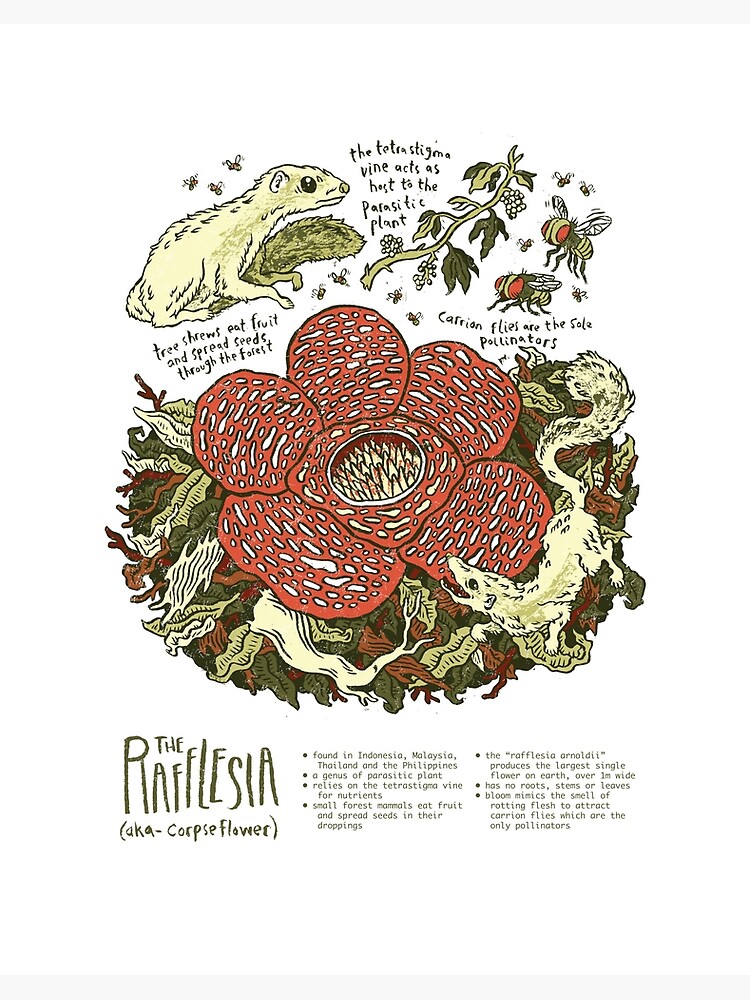This poster, with its charming, cartoon-like design, vividly illustrates the unique life cycle of the Rafflesia, known commonly as the corpse flower. Dominating the center of the image is a striking portrayal of the corpse flower, depicted with large red petals adorned with white spots, and a central cavity ringed by spikes. Surrounding the flower are various elements of its ecosystem: 

- At the top of the image, amidst lush greenery, a pair of squirrel-like tree shrews are shown. The associated text explains that "tree shrews eat fruit and spread seeds through the forest."
- To the left, a vine with noticeable leaves represents the Tetrastigma vine, the necessary host for the parasitic Rafflesia. The text here reads, "The Tetrastigma vine acts as host to the parasitic plant."
- On the right side, small pollinator flies, identified as carrion flies, are depicted with the description, "Carrion flies are the sole pollinators."

The bottom of the poster highlights the name "Rafflesia, a.k.a. corpse flower," followed by a bulleted list of intriguing facts:
- Found in Indonesia, Malaysia, Thailand, and the Philippines.
- Relies on the Tetrastigma vine for nutrients.
- Small forest mammals consume its fruit and disperse seeds through their droppings.
- Produces the largest single flower on Earth, measuring over one meter wide.
- Lacks roots, stems, or leaves.

Additionally, the flower emits a smell similar to rotting flesh, which attracts carrion flies, its exclusive pollinators. This detailed artistic presentation effectively educates viewers on the fascinating ecology and biology of the corpse flower.